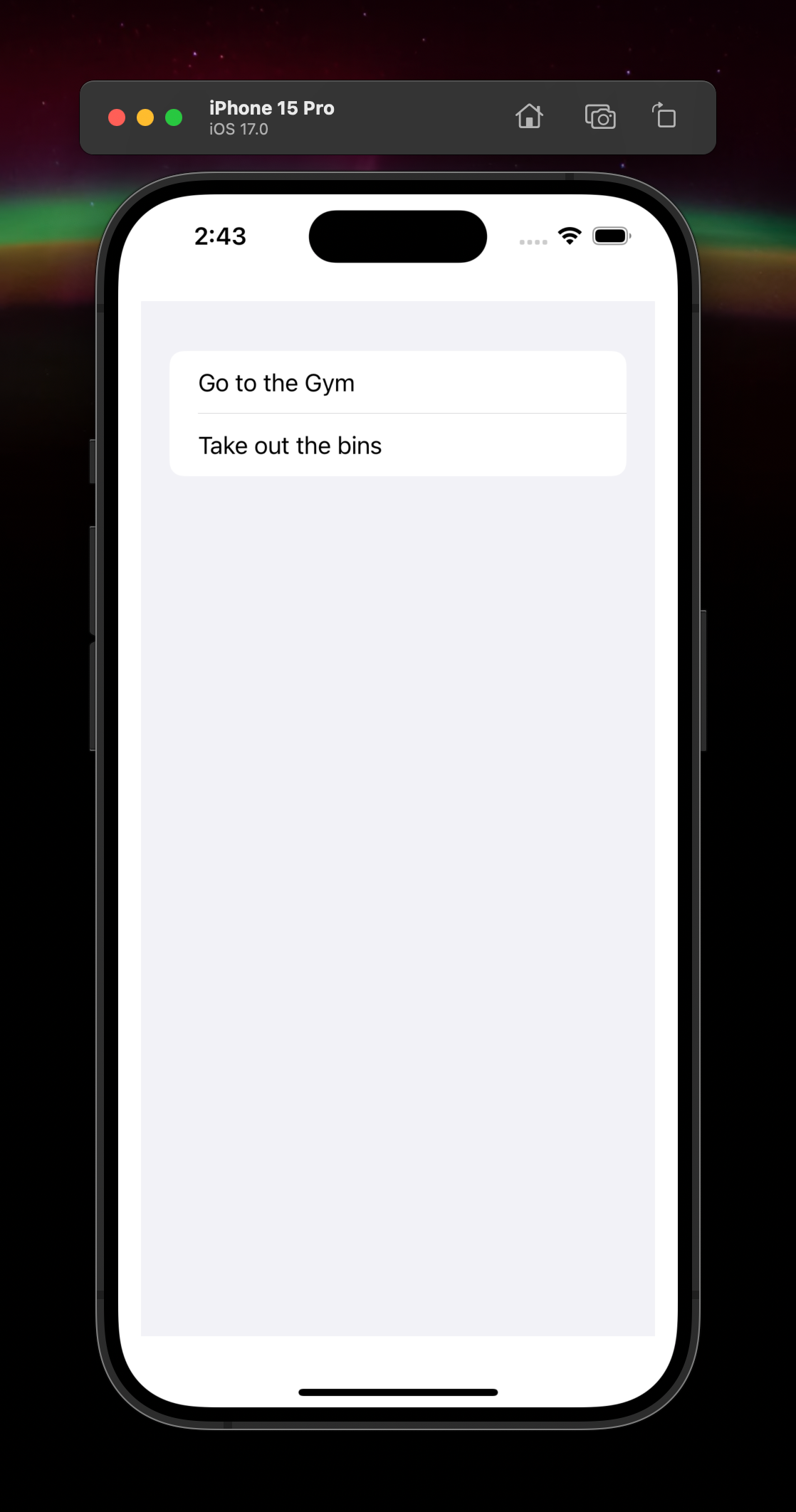The image is a rectangular portrait-oriented photograph, significantly taller than it is wide, with a predominantly black background featuring subtle swirls of green. The background is largely devoid of significant text or imagery except for a slightly lighter rectangle occupying the top portion of the picture.

Within this lighter rectangle are three circles aligned on the left. The first circle is solid red, the second is orange, and the third is green. To the right of these circles, white text reads, "iPhone 15 Pro iOS 17.0." On the far right of this rectangle are three icons: a house, a camera, and a box with an arrow pointing to the right.

The central focus of the image is the iPhone screen, which has a gray background and minimal content. In the top left corner of the screen, the number "243" is displayed, while the top right corner shows a wireless signal icon and an image of an almost full or possibly full battery. Below these icons, two lines of text are present: "go to the gym" and "take out the bins." The remainder of the iPhone screen is blank except for a horizontal line at the very bottom, which is a built-in feature of the iPhone interface.